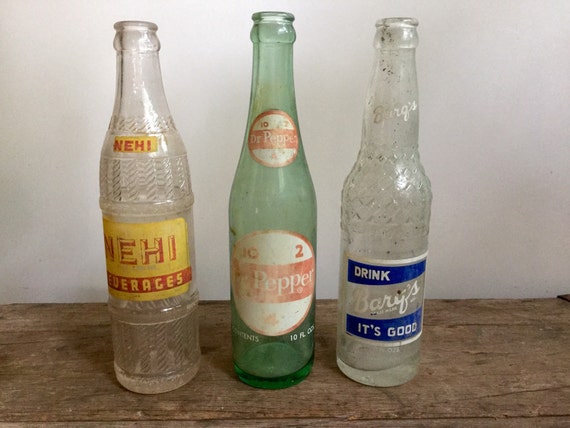This color photograph features three antique glass soda bottles, each distinct in labeling and color, sitting on a wooden surface against a plain white backdrop. The bottle on the far left is a clear glass bottle with a vintage label. At the top, it reads "Nehi" in red letters on a yellow background, followed by a larger yellow label with "Nehi" in red letters and "Beverages" underneath. The middle bottle is a pale green glass bottle bearing two labels. The upper label reads "Dr. Pepper," and the bottom label reiterates "Dr. Pepper" with additional details including "10 fluid ounces." The third bottle on the right is also made of clear glass. At its neck, it says "Barq’s" and features a label divided into sections: a blue top section stating "Drink" in white letters, then a clear middle section with "Barq’s" in white letters, followed by another blue section at the bottom stating "It's Good" in white letters. All three bottles are empty, showing signs of age and dust, enhancing their nostalgic, vintage appeal.